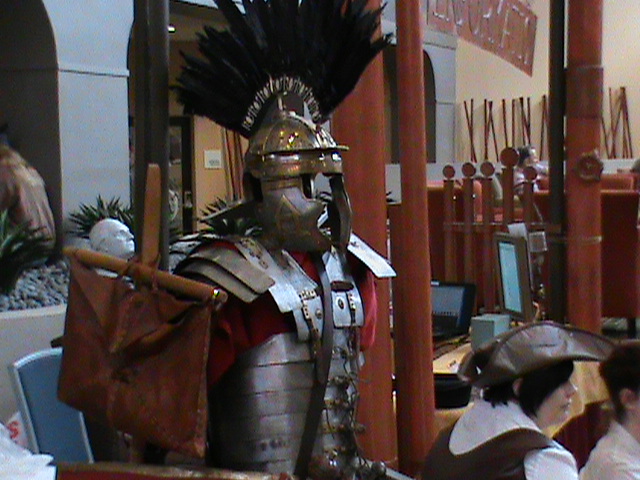The image depicts an elaborate scene centered around a Roman-themed event with a display of intricate armor. The focal point is a suit of armor prominently placed on the left side of the image. This armor, reminiscent of ancient Roman military gear, includes a striking helmet adorned with a mohawk of black feathers. The helmet itself is a mix of bronze and gold metals. The torso features a combination of sturdy metal chest and abdomen plates, all set over a red garment. The armor also includes metal shoulder pads and intricate bands around the waist.

In the background, there's more to the setting—details include red posts and weapons with red or brown handles. Written in gold, though partly obscured, something adorns the red wall behind the armor, which is otherwise black with white sections. Adding depth to the historical ambiance, there's a white statue head looking upward, with several rocks beneath it ranging in shades from brown to beige, and a larger bronze statue to its left. Leafy green elements peek out from among the rocks.

On the right side of the image, two people are engaged in what appears to be part of a historical reenactment or themed village. The foreground features a female wearing a distinctive brown leather hat reminiscent of colonial or old English styles. She has black hair and is dressed in a white undershirt and a brown leather vest. Next to her stands a boy or young man, partially visible, with part of his ear showing – suggesting he might be in his teens.

Adding a modern twist to the historical setting, behind the woman are computer screens that resemble cash registers, hinting at the contemporary nature of the event location, possibly somewhere resembling a museum or an interactive exhibit. Overall, the image melds elements of historical representation with present-day facilities, creating a rich, detailed tableau.